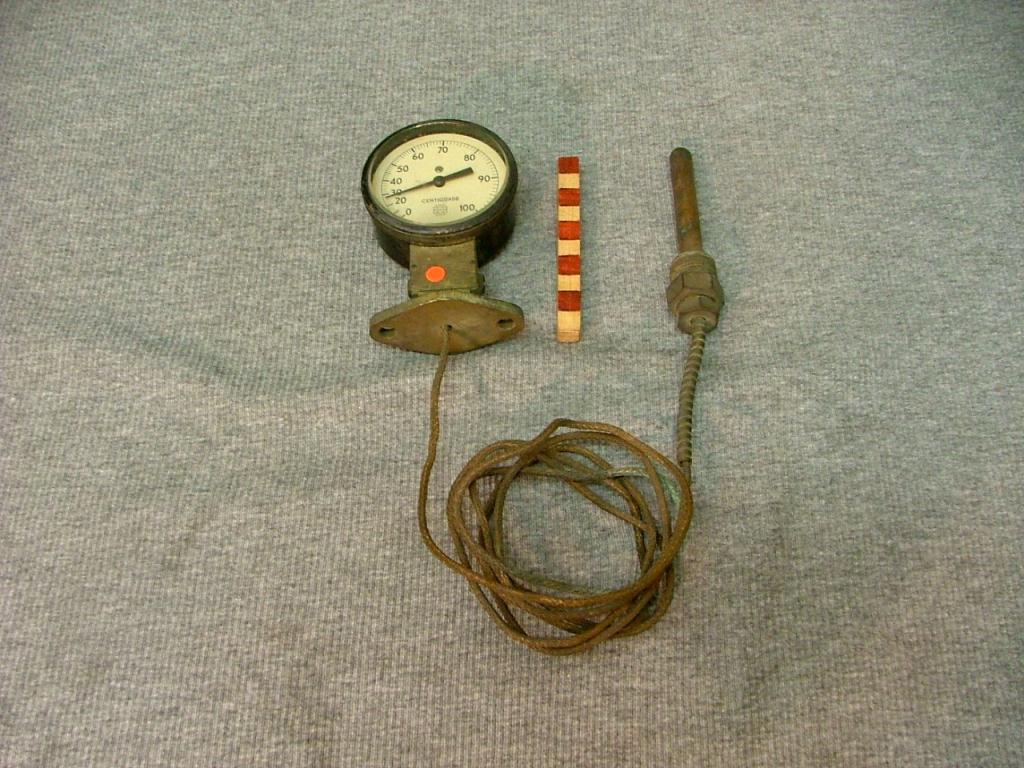A meticulously arranged assortment of vintage machinery is displayed on a richly textured cloth backdrop. The cloth, a soft gray with subtle marbled flecks of yellow and dark gray, features smooth expanses in the top center extending to the corners and puffed-up portions creating intricate ridges in the left center, right center, and bottom left areas.

Prominently centered in the composition is an analog gauge, mounted on a steel base. This gauge has a creamy face encircled by a black rim, and its needle points just shy of the 30 mark on a scale that ranges from 0 to 100. The steel base supporting this gauge includes an orange circle detail and is connected to a lengthy, dark, and slightly grimy wire, which segues into a coiled, thicker wire. This robust wire terminates in a rusted, substantial steel nut and bolt assembly, further extending into a large, dark, and heavily corroded protrusion.

Amidst these mechanical components lies a slender wooden stick, cream-colored and adorned with red-painted square stripes, adding an unexpected touch of color and texture to the scene. The stick is positioned near the middle of the photograph, enhancing the intricate complexity of this compelling still life.